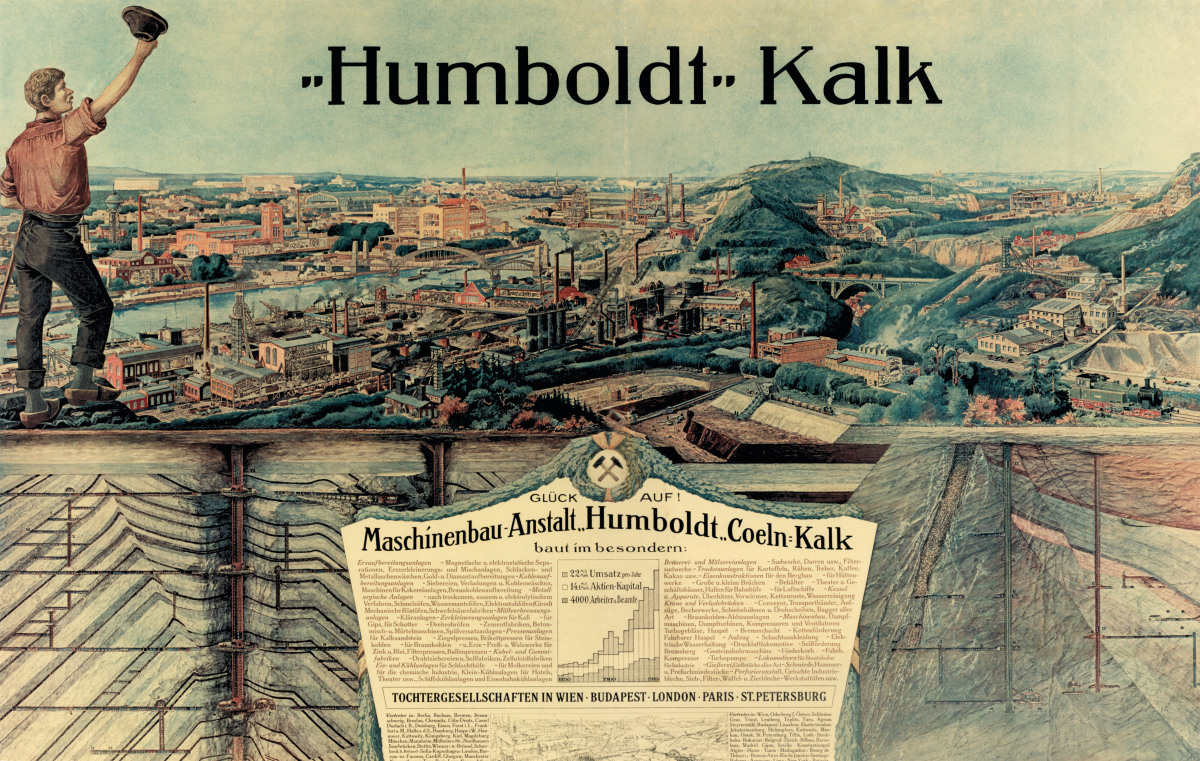The image appears to be a hand-drawn, retro advertisement from the 1940s or 50s, labeled "Humboldt Kalk." The artwork features a man in a reddish shirt, brown pants, and loafers, standing on a rocky outcrop or hillside. He waves his cap in the air while overlooking a small, scenic city nestled in hilly terrain. The detailed background depicts a cityscape with numerous factories, buildings, and infrastructure, including a suspension bridge spanning a river, and a train passing through town. The city's name and various details, such as "Budapest, London, Paris, and St. Petersburg," suggest a rich historical context. An intriguing element at the bottom portrays the inside layers of a mountain, accompanied by a newspaper article or monument in black and off-white tones, written in a foreign language, denoting places like "Maschow" and "Upholt."